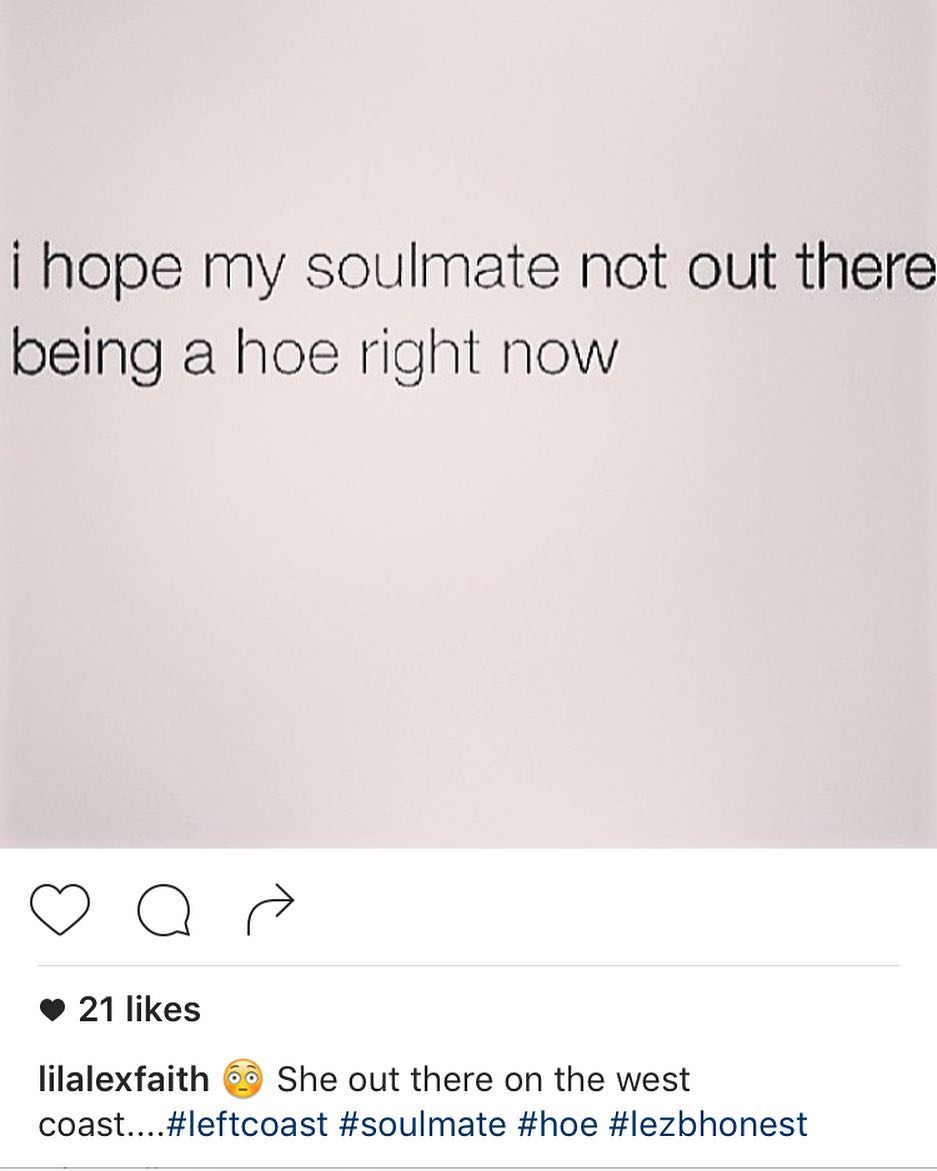The image is a screenshot of an Instagram post featuring a square graphic with a buff beige background. In the center of the square, there is black text written in all lowercase letters stating, "i hope my soulmate not out there being a hoe right now." Beneath this square, the screenshot includes the Instagram interface on a white background. Aligned horizontally to the left are icons in black: a heart outline, a comment bubble outline, and an upward-right arrow. Below these icons, there is a small horizontal line, under which is text prefaced by a solid black heart that reads, "21 likes." Further down, the username "LIL ALEX FAITH" appears, followed by a blushing smiley emoji and the text, "she out there on the west coast... #leftcoast #soulmate #hoe #lezbhonest." The hashtags are displayed in blue text. The overall aesthetic is simple with a limited color palette, emphasizing the black and beige tones.